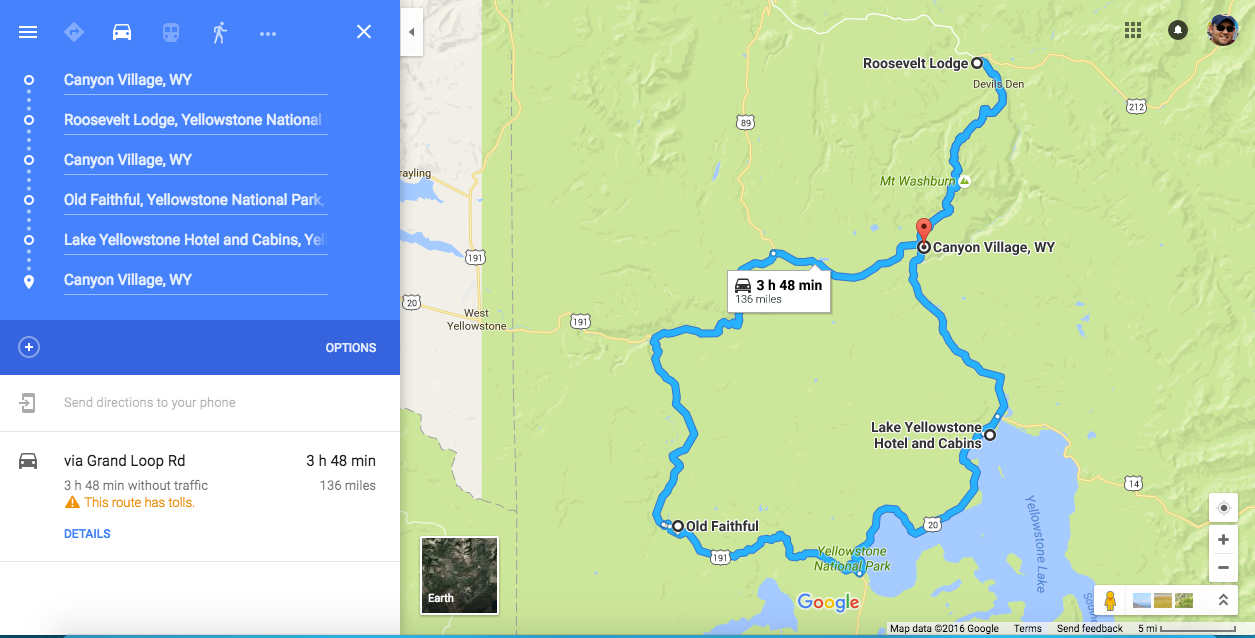This image is a screenshot from Google Maps displaying a detailed travel route in Yellowstone National Park. On the left side, there is a list of significant waypoints: Cannon Village, Wyoming; Roosevelt Lodge, Yellowstone National Park; Old Faithful, Yellowstone National Park; and Lake Yellowstone Hotel and Cabins. The list repeats Cannon Village, Wyoming multiple times, indicating key points along the journey. Beneath the list, an icon of a car is visible, next to a label reading "Grand Loop Road." The travel details specify a duration of 3 hours and 48 minutes covering a distance of 136 miles.

The right side of the image showcases a map with a green backdrop, highlighting the route in blue. This line visually represents the trip through the park, connecting the listed locations. At the bottom of the image, several utility icons from Google Maps are displayed, although their specific functions are not detailed in the screenshot.